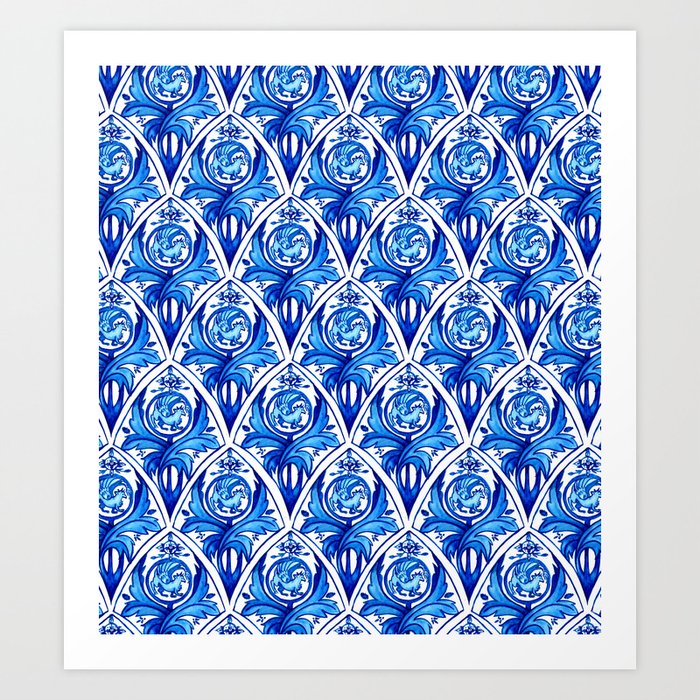The image depicts a detailed blue and white pattern, reminiscent of a wallpaper design. The central motif is framed by white borders and features two distinct shades of blue. Dominating the pattern are diamond shapes characterized by curved sides— the lower edges curving inward while the upper edges protrude outward. Within each diamond, two blue leaves intersect in an X-like formation, and in the space between these leaves at the top, there appears to be a circular shape resembling a horse. Triangular shapes with softened edges are also present, some appearing almost egg-like due to the curved lines. The pattern is notable for its overlapping elements and intricate, animated look, set against a subtle gray background that accentuates the blue and white hues.